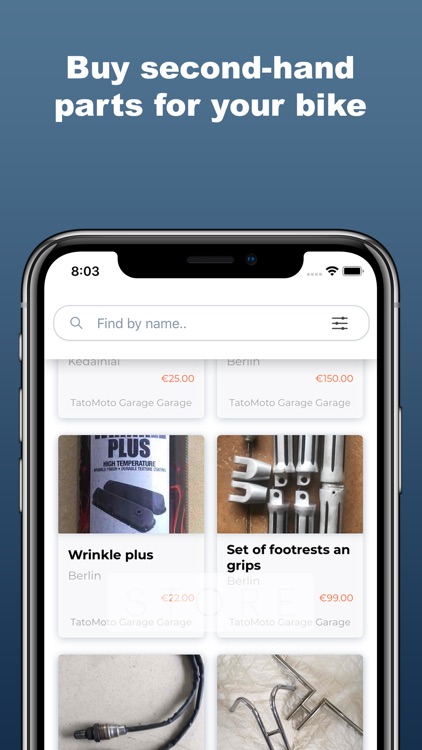The image depicts a detailed advertisement for a website specializing in secondhand bike parts. The background gradient transitions from a light blue at the top to a darker blue at the bottom, creating a visually appealing backdrop. At the very top, in bold white text, the ad reads, "Buy Secondhand Parts for Your Bike."

Central to the ad is an image of a black iPhone, noticeable by its sleek black trim and possibly silver buttons on the sides. Prominently visible are the volume and silence buttons on the left, and the lock screen button on the right. At the upper part of the iPhone's screen, a thick black banner houses the camera hole and the central voice speaker.

Displayed on the iPhone screen is a white-background application interface. The top-left corner shows the time as 8:03, while the top-right corner indicates no cellular signal but shows full Wi-Fi connectivity and battery life. Below this information, a search bar with a magnifying glass icon invites users to "Find by Name." 

Further down, the screen reveals a series of listings organized in six square sections, each representing a product. Although the top two listings are slightly cut off, the visible parts show:

1. A product priced at 25 euros from Tatomoto Garage.
2. Another listing from Berlin marked at 150 euros, also from Tatomoto Garage.

In the middle of the screen are two more prominent listings:

1. An item labeled "Wrinkle Plus" from Berlin, priced at 22 euros with a visual that includes a white label and black objects.
2. A set of gray plastic bike parts for footrests and grips marked at 99 euros from Berlin, again from Tatomoto Garage. It’s noted the word "and" is abbreviated as "A-N," with an extraneous space following the "D."

At the bottom:

1. A listing showing a black cable with a silver spark plug component.
2. H-shaped metal rods depicted in the image of the last listing.

All product prices are displayed in orange, emphasizing the cost alongside the detailed item descriptions.

This clean and detailed organization of the advertisement encapsulates the essentials a potential buyer might look for, highlighting the ease of searching and the variety of secondhand bike parts available.